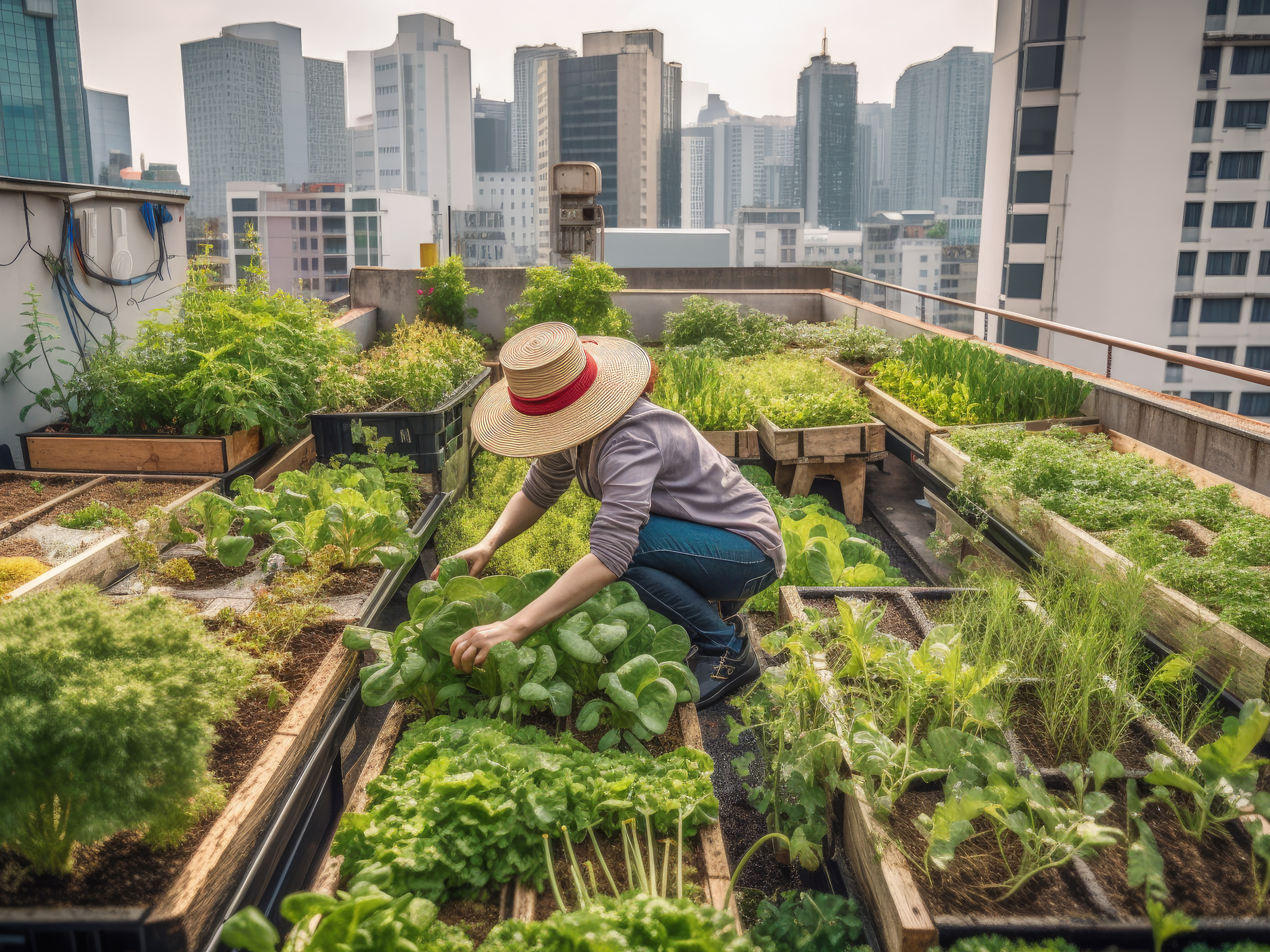The image captures a rooftop garden surrounded by tall city buildings under a smoggy gray sky. There are numerous wooden raised garden beds occupying the space, filled with a diverse array of plants—possibly dill, carrots, radishes, and beans. Amidst these garden beds, near the center of the image, a Caucasian woman with red hair tied in a ponytail is kneeling. She wears blue jeans, dark shoes, and a purple long-sleeved shirt rolled up to her elbows, along with a straw hat featuring a red band. Her face is not visible, as she is focused on tending to a leafy plant in front of her. The rooftop area is encircled by a short metal railing, with visible cables along the side, adding to the urban atmosphere of this unique garden space.